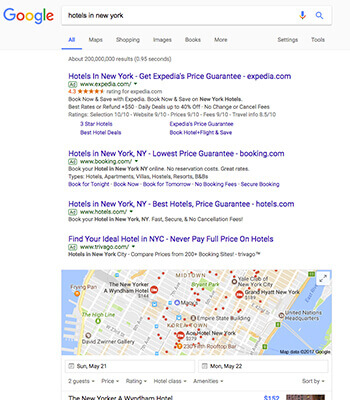The image is a screen capture of Google search results for "hotels in New York." The search query is clearly visible at the top of the page. Below the search bar, the central portion of the screen displays several search results, each promoting hotel booking services with price guarantees. The first result advertises Expedia's price guarantee. Following it, the second result highlights Booking.com's lowest price guarantee for hotels in New York, New York. The third entry is from Hotels.com, offering the best hotels with a price guarantee. The fourth result is from Trivago, encouraging users to find their ideal hotel in New York without paying full price.

The lower third of the page features a detailed street map of lower New York, extending from the left to the right edge of the screen. This map includes pinned locations of various hotels such as The New Yorker and Grand Hyatt New York, as well as notable landmarks like the Empire State Building. Additionally, two date fields are visible below the map, one indicating "Sunday, May 21" on the left and the other marked "Monday, May 22" on the right.